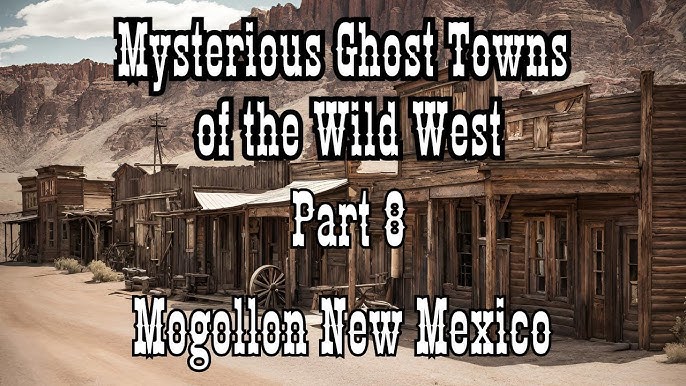The image is a vintage poster dominated by beiges, greys, and browns, depicting a street scene from the Old West. The one-block-long street is lined with wooden buildings constructed from logs, featuring simple doors, windows, and porch coverings supported by tall logs. On the right side, a detailed view reveals a wagon wheel leaning on one of the buildings, adding to the historical ambiance. In the background, brownish-reddish mountains and canyons rise against a greyish sky with a single fluffy white cloud. Overlaid on the photograph is white text outlined in black, written in a Western font. The text reads: "Mysterious Ghost Tours of the Wild West, Part 8, Mogollon, New Mexico." This visually compelling poster evokes the rugged atmosphere of the era and sets the theme for a historical ghost tour.